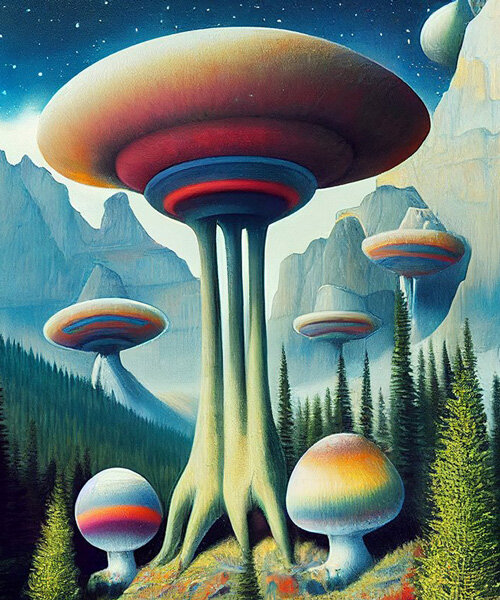Set against a backdrop of a towering mountain range, this digitally rendered sci-fi painting exudes an organic-meets-inorganic aesthetic that alludes to a fantastical world. The sky above, dotted with stars, casts a serene blue hue over the landscape. Dominating the foreground are towering structures that appear to be a fusion of trees and mushrooms. The most prominent one features a blue base with branching, tree trunk-like legs supporting a multi-colored, UFO-style disc at its top, shimmering in shades of red, yellow, and green. This main structure emanates an almost otherworldly presence as it seemingly grows from the forest floor. 

Surrounding it are smaller, round, and vibrant mushroom-like formations in hues of yellow, red, and green, littering the grassy terrain like alien flora. The scene is further accentuated by dense clusters of pine and evergreen trees, stretching down into a verdant valley. In the distance, additional mushroom-like constructions continue the theme, including one that boldly crowns a mountain peak. The overall impression is that of an alien planet or fantasy realm, rich in detail and color, perfectly suited for the cover of a captivating sci-fi paperback.